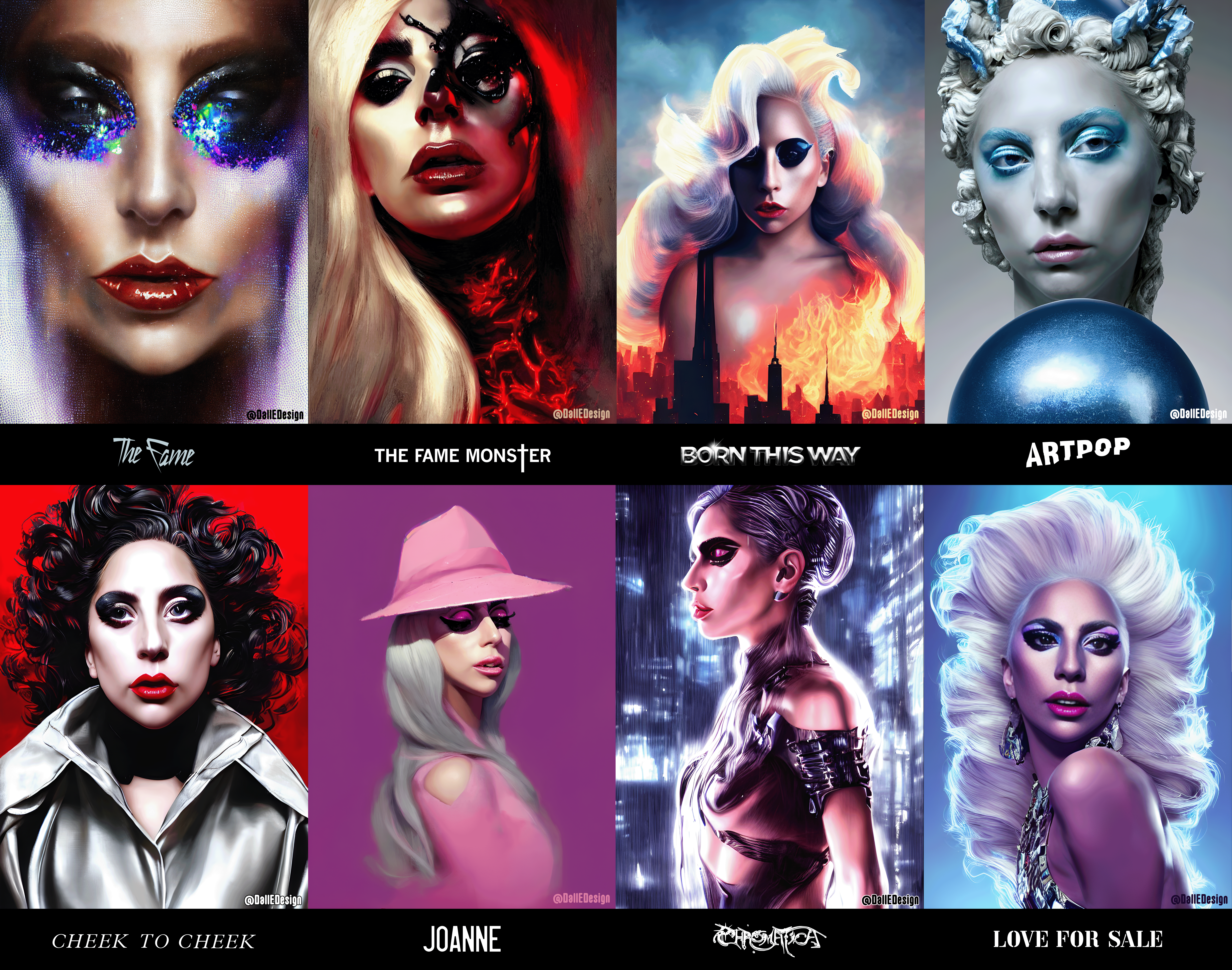The image is a compilation of eight album covers of Lady Gaga arranged in two rows, each featuring a distinctive look or style. The top row includes "The Fame," showcasing a close-up of Lady Gaga's face with thick glitter eyeshadow, "The Fame Monster" with a high-tech steampunk eyepiece over her left eye, "Born This Way" depicting her torso emerging from a burning city skyline, and "Art Pop," portraying her as a statue with white, curly stone hair and blue accents. The bottom row starts with "Cheek to Cheek," where Lady Gaga appears with long wavy hair and a grey top, followed by "Joanne," featuring her in a pink outfit and hat, and a side profile image with unreadable font resembling 'Photopia,' displaying her in fantasy armor. The last image is "Love for Sale," where she strikes a glamorous pose reminiscent of Marilyn Monroe, wearing a shiny dress and looking over her shoulder. All the images are bright, vibrant, and showcase Lady Gaga in various costumes and makeup, emphasizing her diverse and eclectic style.